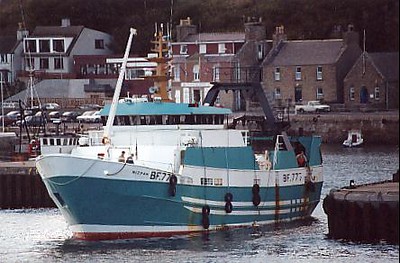The image captures a medium-sized, blue-green and white commercial ship in a bustling, well-built harbor. The ship, which bears the markings "BF777," appears worn and rust-stained, evoking a sense of age and history consistent with vessels from the 1950s or 60s. Black tires hanging from chains along its sides contribute to its rugged appearance. The boat is emerging from the dock area, suggesting recent or imminent activity. In the background, a collection of brown brick buildings with white accents, likely part of a mixed residential and commercial area, frame the scene. Additional boats and various cars are visible, enhancing the sense of a busy, functional port. The overall setting conveys a slightly aged and weathered charm, with an impression of constant movement and industry.